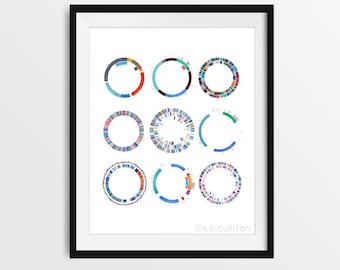The image depicts a photograph of a small framed painting or chart mounted on a white wall. The frame is a thin black rectangle, and within it lies a white central background featuring a grid of nine colorful circles, arranged in three rows and three columns. Each circle is distinct, showcasing a variety of vibrant colors including red, blue, green, yellow, and orange, with some circles displaying multi-colored patterns and others having segmented or dotted designs. Despite their small size, the circles are clearly vibrant and are uniformly aligned in the frame. The absence of explanatory text or additional objects emphasizes the colorful patterns as the focal point of the image, which is captured in bright, natural lighting, adding to its clear visibility and detail.